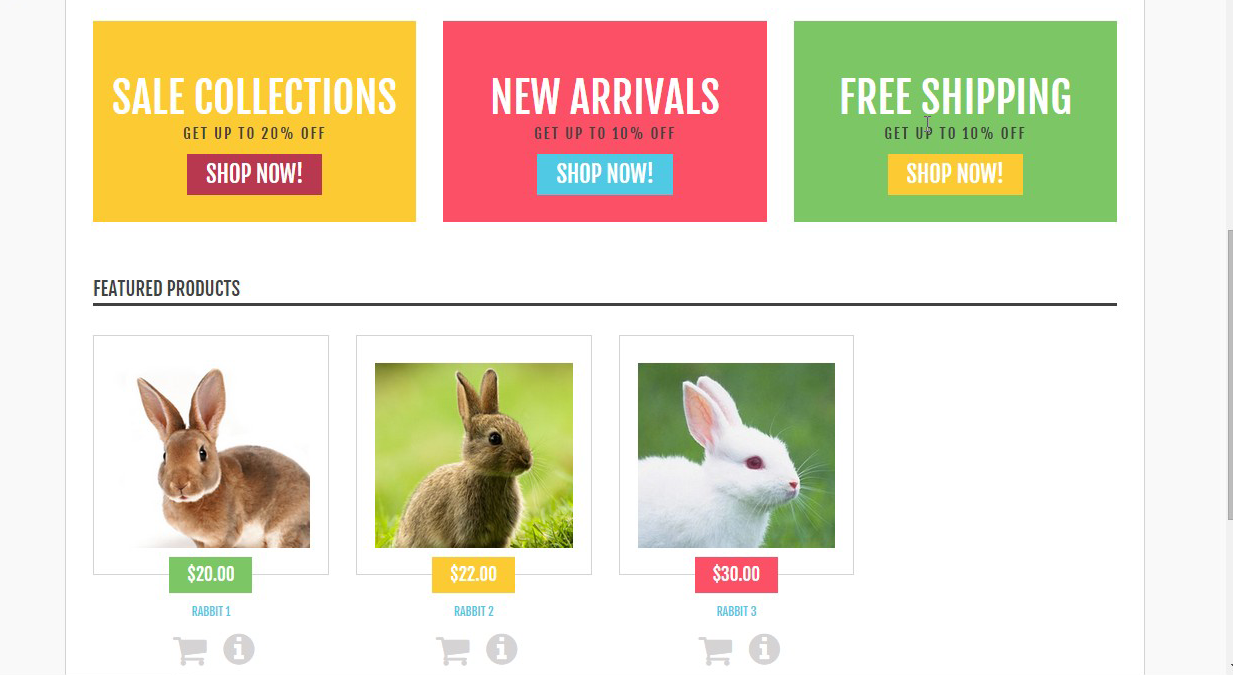**Webpage Design - Promotional Section and Featured Products**

The webpage is under the "Website" category, featuring a minimalistic layout with various promotional offers and product displays. 

At the top left corner, there is a grey border with a highlighted yellow box. This box contains the text "Sale Collections" in white letters and smaller text below it, "Get up to 20% off," in black letters. Beneath this yellow box, a red button prominently displays the words "Shop Now!"

To the right of the yellow box, there is a pink box with the text "New Arrivals" in white letters and a smaller black text below it, "Get up to 10% off." Underneath this box, a teal-colored button reads, "Shop Now!"

Adjacent to the pink box is a green box with "Free Shipping" in white letters, followed by smaller black text underneath stating, "Get up to 10% off." This green box is paired with a yellow button below that says "Shop Now!" in white letters.

The webpage also features three distinct products:

1. **Rabbit One**: Priced at $20, this product showcases a plump, adorable rabbit with a cute face. The rabbit possesses a white belly and brown fur, but its paws are not visible in the image. A green box beneath the picture indicates the price.

2. **Rabbit Two**: This item is available for $22 and features a slimmer rabbit seated on the grass. It is smaller in size, somewhat akin to a squirrel, and has brown fur. The green price box is situated below the image.

3. **White Rabbit**: The premium product, costing $30, displays a white rabbit with pink ears basking in the sunlight. The green price box below the image states its price.

These detailed sections and products aim to capture the attention of potential buyers with clear and attractive offers.